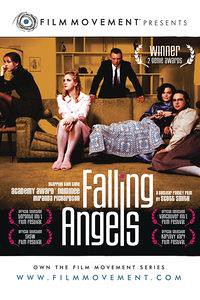This image appears to be a low-resolution movie poster, depicting the cover of a film titled "Falling Angels." The scene showcases a group of five people—men and women—arranged around a tan or gold-colored couch that overlaps with a similarly hued rug and wall, creating a cohesive monochromatic backdrop. At the top of the poster, the text reads "Film Movement Presents," and an award emblem in the right-hand corner suggests the film has received independent accolades. The arrangement of the individuals includes a man in a black suit leaning against the couch, two women seated on it, one on the armrest, and another woman resting on the floor against the couch. The couch appears saggy or well-used, with one woman on the right side having a blanket over her legs. Below the image, in large white letters, the title "Falling Angels" is prominently displayed, followed by the statement "Own the Film Movement Series" and a website link, www.filmmovement.com.